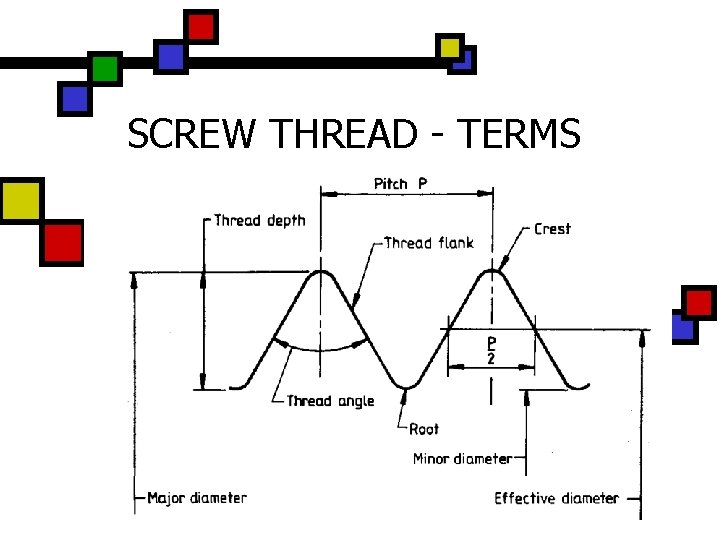This image is a detailed diagram titled "Screw Thread Terms" located beneath a thick black line adorned with multi-colored squares including blue, green, red, and yellow. To the left of this title, there are additional red and blue squares. The chart at the bottom features black lines and curves, representing peaks and troughs akin to hills or mountains, labeled with various screw thread terminology. Key terms identified in the diagram include thread depth, thread angle, pitch P, thread flank, root, major diameter, effective diameter, minor diameter, and crest. The overall visual layout appears ideal for educational purposes, possibly used in a setting that requires understanding of screw thread mechanics or in a maintenance context.